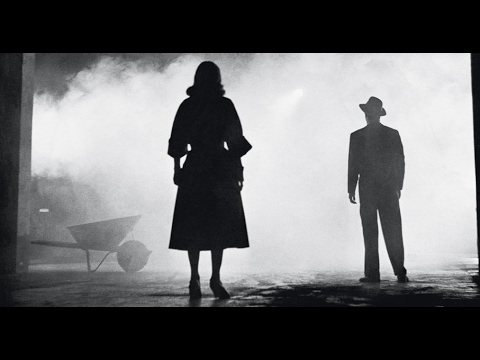In this black-and-white photograph, likely taken from an old movie, two figures are depicted in striking silhouette form. Centrally positioned, the woman, donned in a vintage dress and heels, faces the man, who sports a suit and a hat tilted to the side. The man stands slightly to her right, seemingly looking at her, creating a scene rich in implied narrative. Both figures are enveloped in mist or fog, adding a layer of mystery and atmosphere. To the left of the woman, a wheelbarrow is faintly visible, enhancing the old-fashioned, possibly rural setting. The overall image exudes a sense of mid-20th-century nostalgia, with the black background and silhouetted figures reminiscent of a dramatic moment frozen in time.